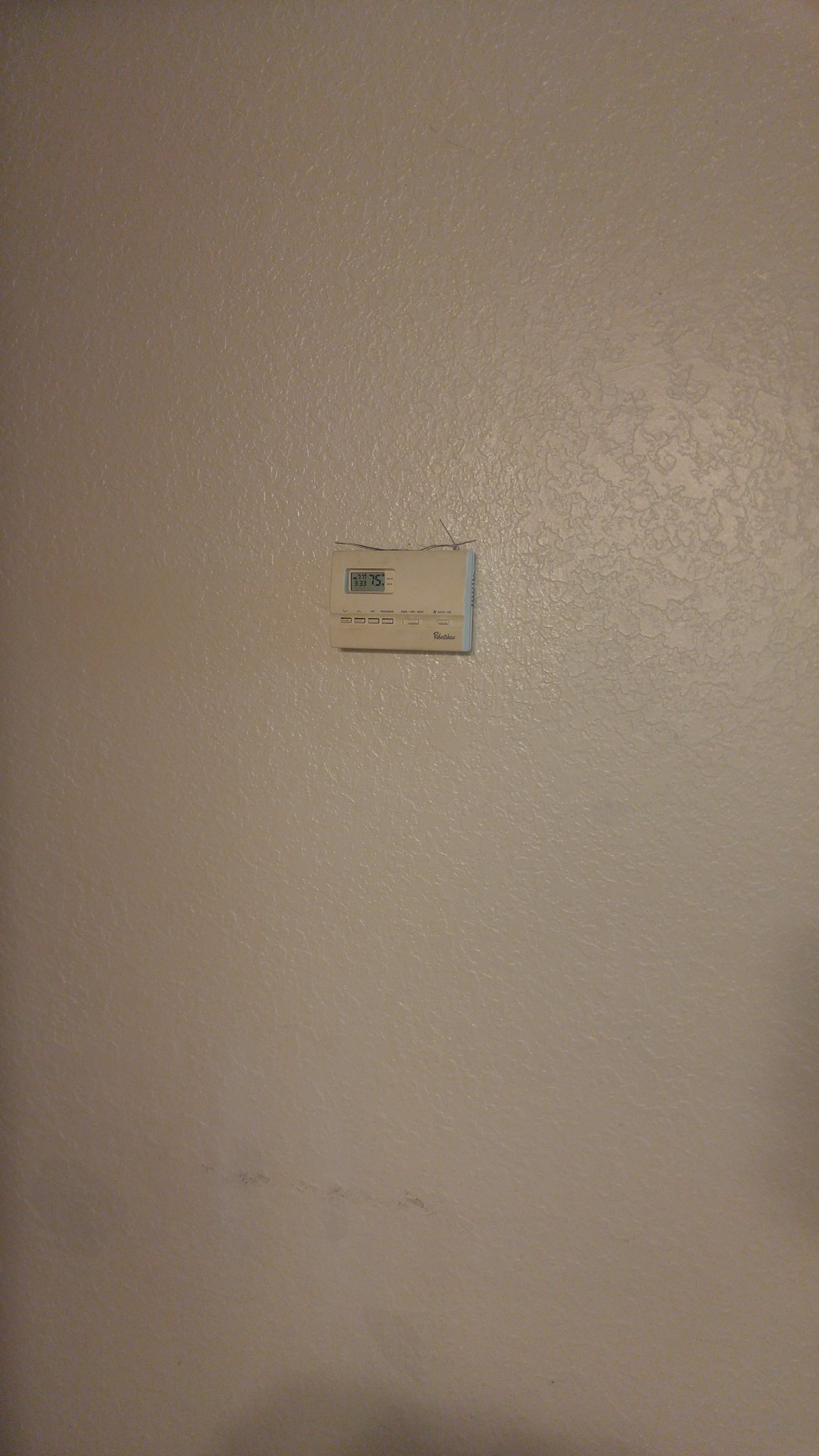A simple yet evocative photograph presents a vertically oriented image focusing on a vast, textured white wall. Dominating the center of this expansive backdrop is a small, outdated analog thermostat with a clunky interface. The thermostat features a tiny screen that displays the temperature without any backlighting. The wall itself exhibits a textured finish, resembling a popcorn or stucco surface, offering a tactile richness that would be undeniable to the touch. Below, a faint, lumpy shadow suggests the presence of the photographer, subtly hinting at light coming from behind. The overall composition is stark, with the large wall amplifying the minimalist and somewhat nostalgic presence of the small thermostat.